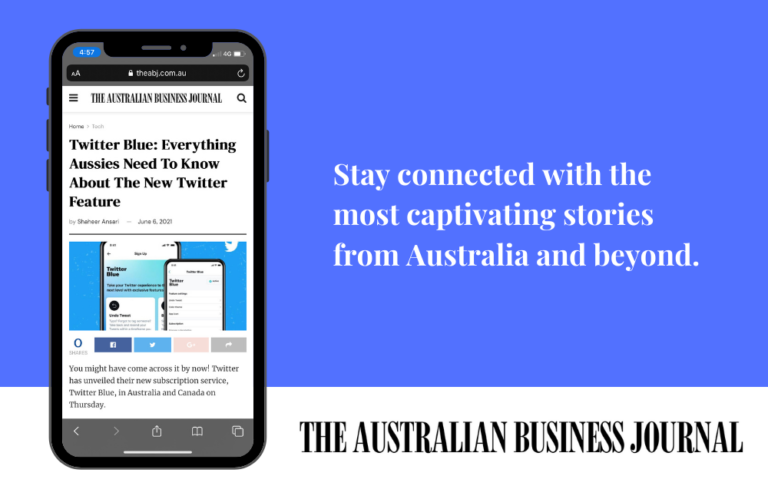The advertisement for the Australian Business Journal features a predominantly purple background, covering approximately 80% of the page, with the bottom section in white. On the right side of the purple background, a text proclaims, "Stay connected with the most captivating stories from Australia and beyond." Adjacent to this text is an image of a black iPhone displaying a page from the Australian Business Journal. The screen showcases a news article titled "Twitter Blue: Everything Aussies Need to Know About the New Twitter Feature" with an accompanying smaller image depicting two phones. Anchoring the design, the white section at the bottom of the ad prominently features the publication's name in bold, black, capitalized letters: "THE AUSTRALIAN BUSINESS JOURNAL." The ad effectively highlights the journal's mobile accessibility and engaging content.